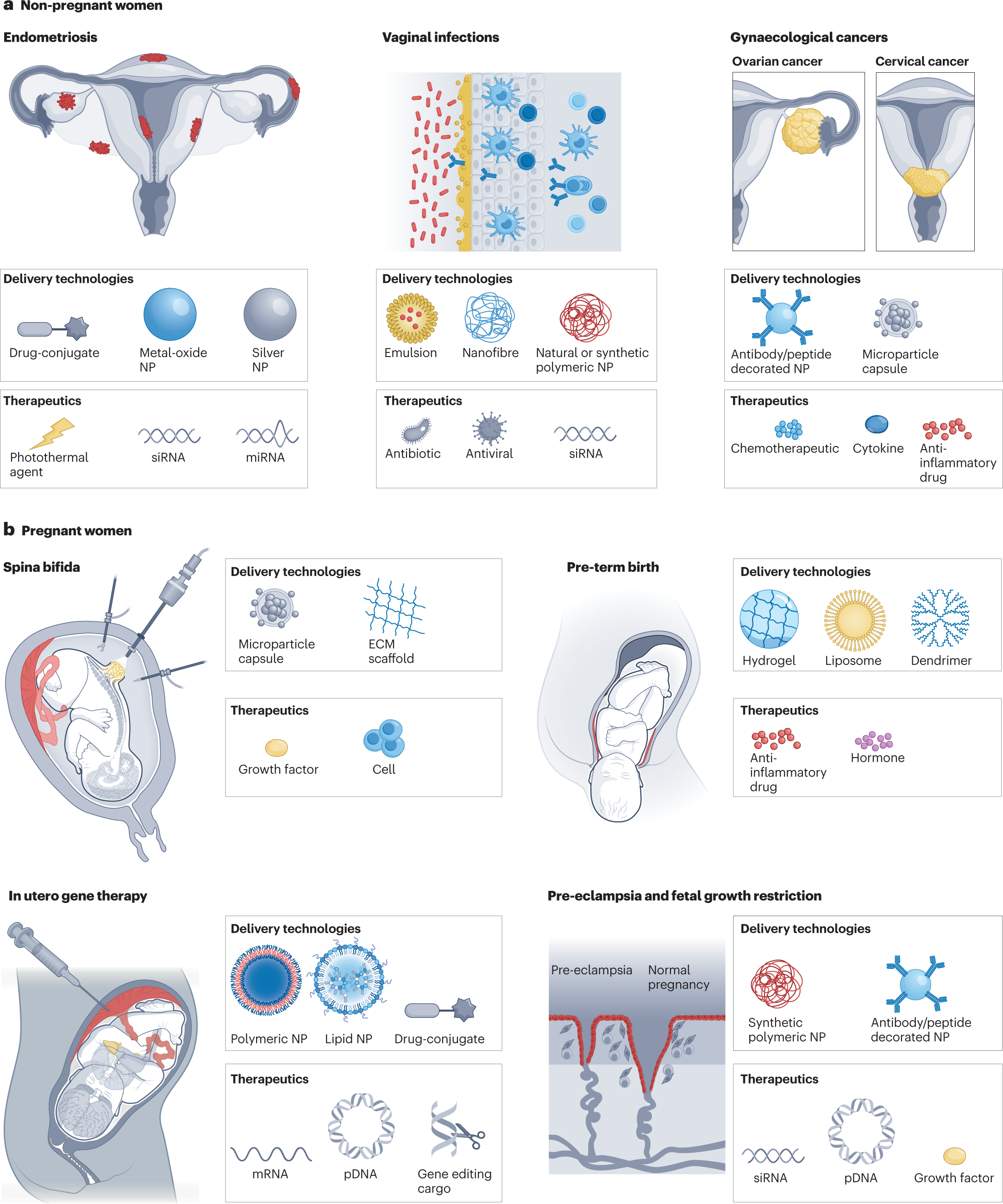The image is a detailed set of seven diagrams illustrating various conditions and infections of the uterus, complete with treatments and delivery technologies. The diagrams encompass endometriosis, vaginal infections, gynecological cancers, spina bifida, preterm birth, in utero gene therapy, and eclampsia and fetal growth restriction. Each section depicts detailed illustrations of the specific organs affected, showcasing conditions such as endometriosis with red spots, vaginal infections with multicolored bacteria, and gynecological cancers in the fallopian tubes and cervix. Accompanying each diagram are sections on therapeutics and delivery technologies, outlining specific medicines and techniques used for treatment. Flashy red, blue, and yellow elements highlight important details within each gray-toned diagram, enhancing the visual representation of the cellular and genetic interactions pertinent to each condition.